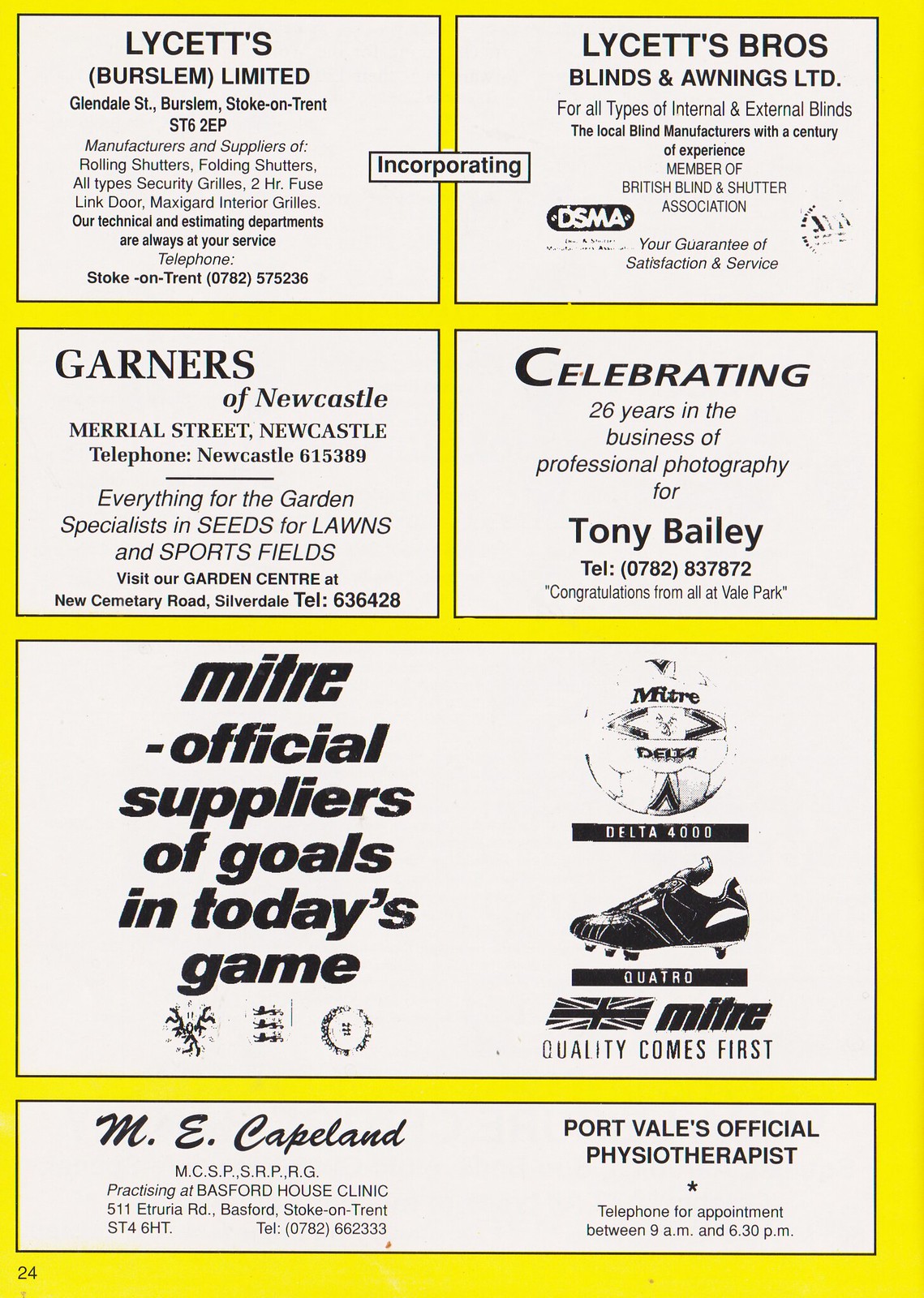The image appears to be a yellow page from a booklet, with several white rectangular advertisements and the number 24 in the bottom left corner. Starting from the top left, the first ad reads "Lysette's of Burslem Limited" with small fine print related to security grills, folding shutters, and similar products. Adjacent to it on the right, the next ad is for "Lysette's Bros Blinds and Awnings Ltd," detailing various internal and external blinds. Centrally between these, there is a smaller box simply stating "incorporating."

Moving down, on the left side is an ad for "Gardner's of Newcastle" located on Muriel Street, specializing in garden supplies, including seeds for lawns and sports fields. To the right of this, an ad celebrates "26 years in the business of professional photography for Tony Bailey," complete with a phone number and congratulations from all at Vail Park.

Dominating the lower half of the page is a larger advertisement for "Mitre, Official Suppliers of Goals in Today's Game," featuring images of a soccer cleat and ball. Finally, at the very bottom, there's an ad for "M.E. Copeland, Port Vale's Official Physiotherapist."

Overall, the page showcases various business sponsors, each clearly marked in black font within individual white boxes, all set against a vibrant yellow backdrop.